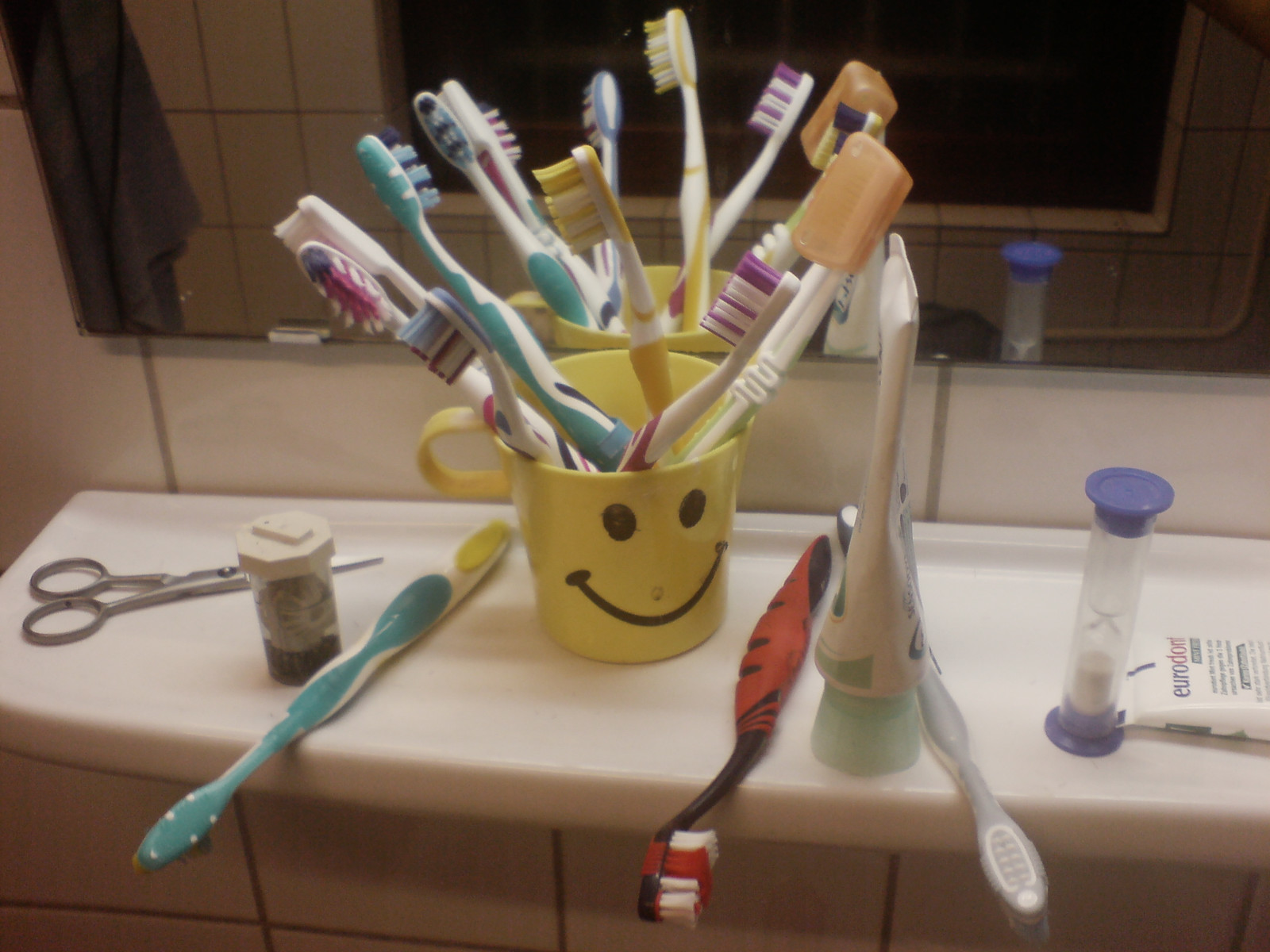In this slightly grainy photograph taken in a dimly lit bathroom, a rectangular mirror spans the top third of the image, reflecting a dark window and possibly a hanging towel. Below the mirror extends a white porcelain shelf, adorned with various items. Dominating the center of the shelf is a cheerful yellow cup with a smiley face, brimming with a collection of colorful toothbrushes, including one with an orange bristle cap. Scattered on the shelf are three additional toothbrushes, their bristles pointing towards the viewer. To the left of the smiley cup, there is a pair of silver scissors and a cylindrical container, possibly holding contact lenses, while a thin tube of toothpaste stands to the right. Further to the right, a small sand timer completes the collection on the ledge. The background reveals white square tiles, characteristic of a typical bathroom setting.